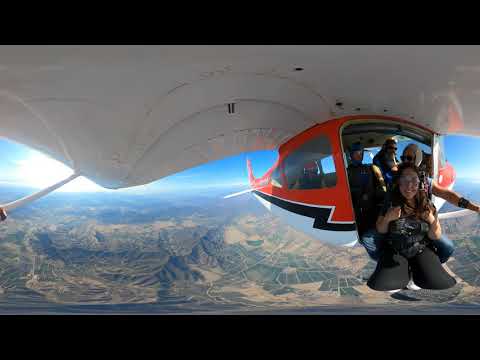In this highly distorted fisheye panoramic image, a red and white airplane with a distinct black lightning bolt dividing the colors captures attention against a backdrop of clear blue skies. The airplane appears compact due to the curved lens effect, with the tail clearly visible on the left. Above the plane, off-white wings and struts come into view, framing a bright source of white light. Below, and stretching into the distance, a patchy landscape of green and brown segmented fields and rocky terrain is seen from a high altitude.

Inside the plane, three helmeted individuals are visible, with a pilot wearing sunglasses positioned towards the cockpit. In the foreground, a woman with goggles and black spandex clothing seems to defy gravity, appearing to sit outside the plane with knees bent and hands gripping parachute straps, her joyful expression aimed towards the camera. This surreal effect makes it appear as though she is suspended on air, ready to jump. The image captures a thrilling moment of anticipation and adventure, blending the serene expanse below with the dynamic action of skydiving preparations above.